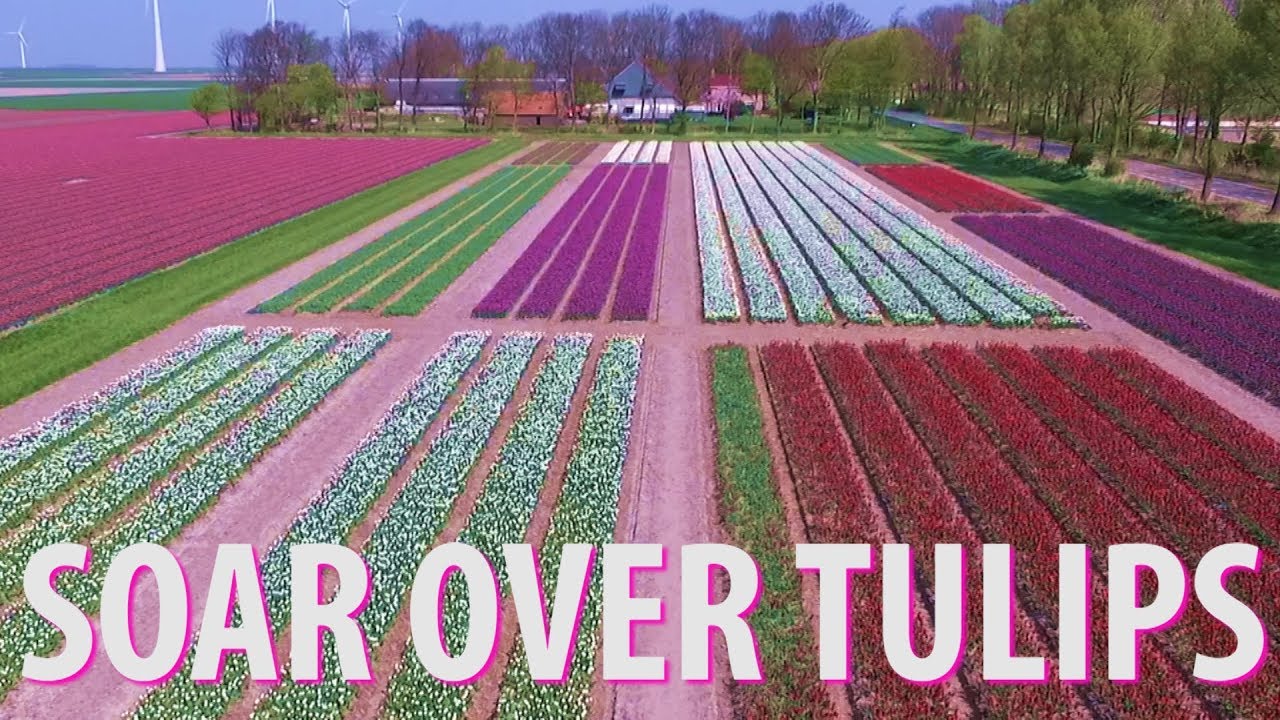In the bright afternoon light, a stunning photograph captures a well-maintained flower field, reminiscent of Amsterdam’s famous tulip fields. The scene is dominated by vibrant rows of tulips in multiple colors, creating a mesmerizing spectrum across the expansive landscape. Stretching over the left side are wide swathes of pink tulips, adjacent to a neatly trimmed row of green grass. Towards the bottom left, clusters of white tulips bloom, while the bottom right explodes in vivid reds. The center is adorned with columns of purple and white tulips, seamlessly blending into additional white tulips. Along the right margin, shades of purple, red, and green tulips are framed by a sidewalk bordered with green grass.

In the distance, the horizon is lined with trees and sprinkled with buildings, adding depth to the floral expanse. The top of the image features a clear blue sky, where white windmills gracefully stand, accentuating the picturesque allure. The text "Soar Over Tulips" is boldly inscribed at the bottom, inviting viewers to immerse themselves in this floral paradise. This captivating combination of tulips, greenery, and charming background structures celebrates the breathtaking beauty of nature’s tapestry.